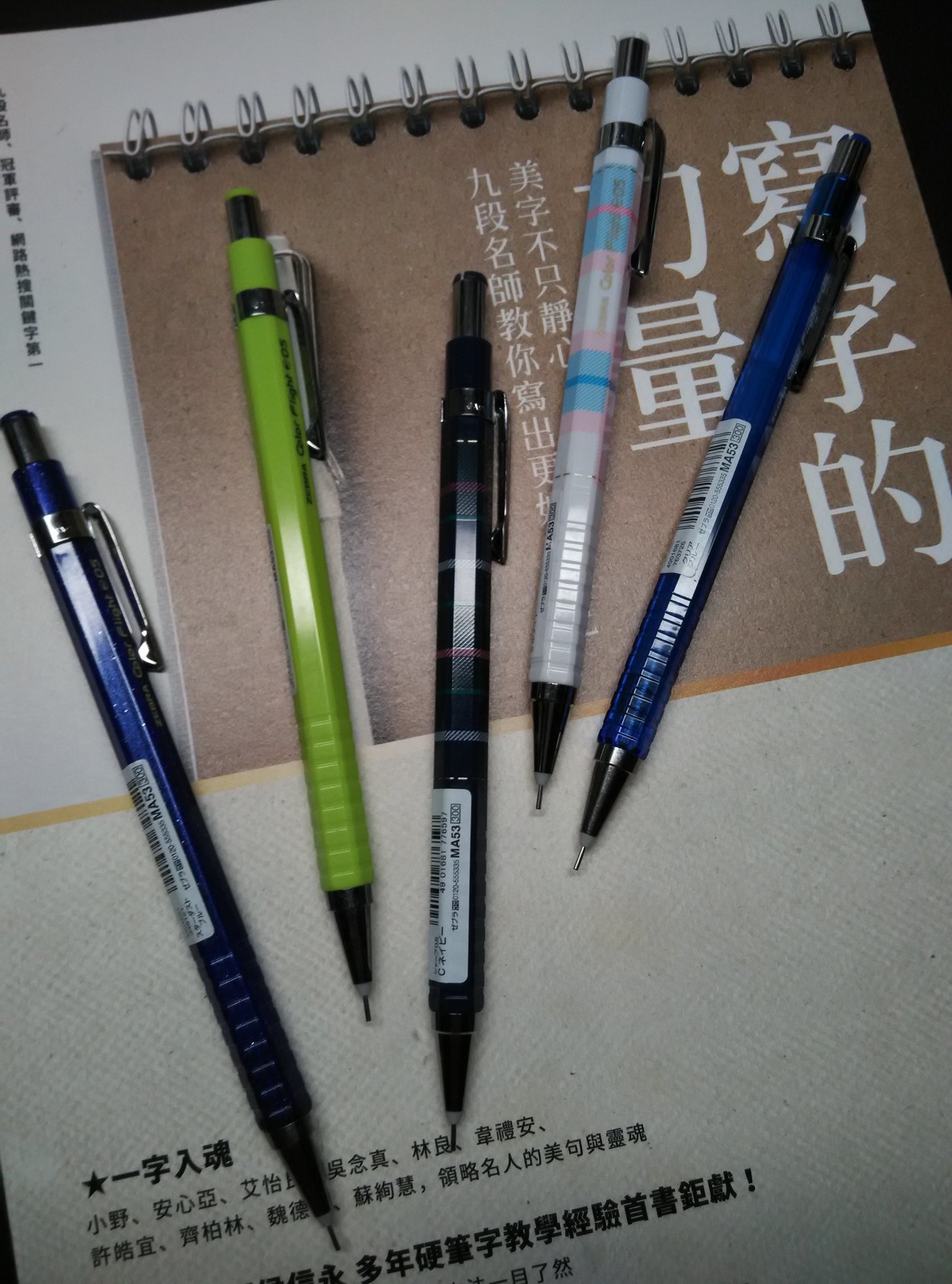This detailed photograph captures a close-up of two pieces of paper adorned with Chinese or Japanese characters rendered in black ink. One of these papers is a brown spiral-bound notebook featuring additional characters in white ink. At the center of the image are five mechanical pencils, meticulously aligned and facing towards the camera. The pencils, oriented from left to right, are colored dark blue, lime green, black with colored stripes, white with blue and pink accents, and dark blue again. Each pencil exhibits a grip texture, a metal clip on the side, and a button at the end opposite the tip. The scene is set against a light gray background from an overhead perspective, showcasing the text and notebook detail in stark contrast. The top corners of the image reveal subtle black background areas on the notebook, further enhancing the prominence of the objects in focus.